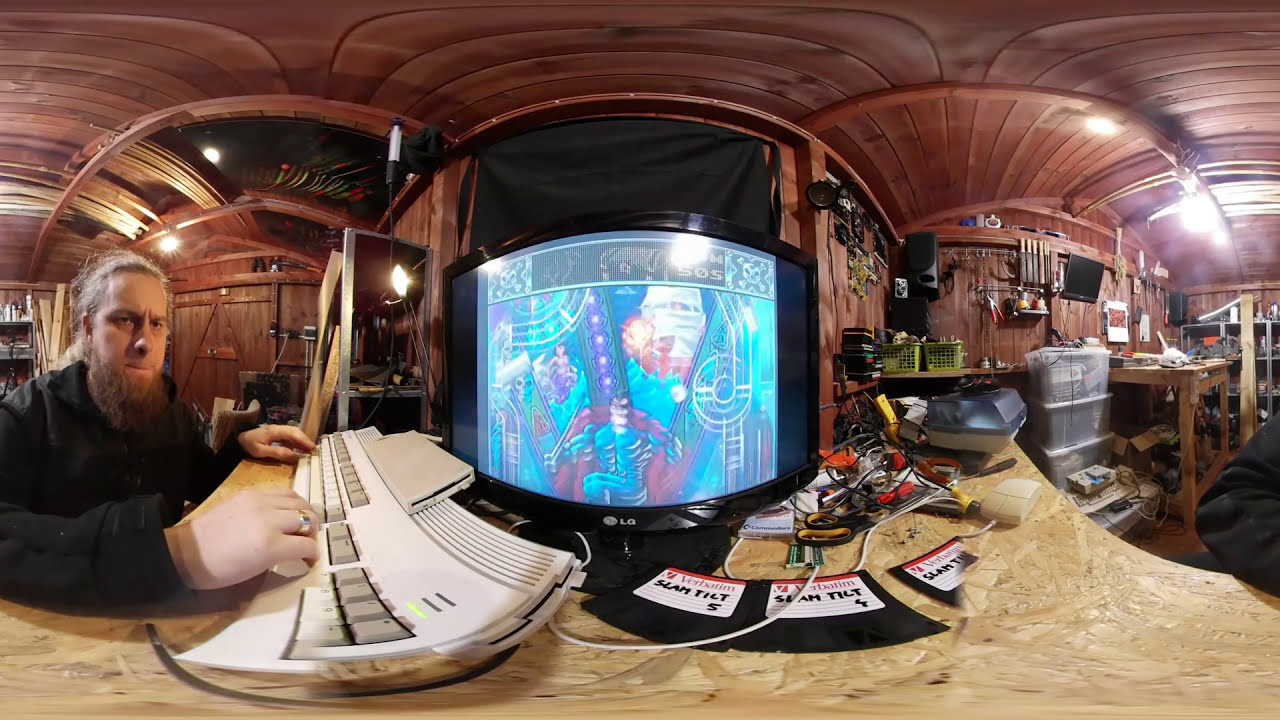In this panoramic, fisheye-lens photograph, a young man with reddish-brown hair and a full beard is intently working at a white keyboard, positioned to the left of the frame. He is dressed in a long-sleeve black shirt and wears a ring on his right ring finger. The setting is a spacious wooden workshop that doubles as a study, with natural light flooding the room. The wooden ceiling and walls add a rustic charm, with various tools and objects neatly organized on shelves and hanging on the wall to the right. In front of the man, a monitor displays a blue-tinted map, possibly a satellite image or video game, and vintage 3.5-inch floppy disks are visible beneath it, evoking a sense of nostalgia. The desk, likely made from compressed wood, is uncluttered except for an unusual disk drive sitting on top of the keyboard, hinting at a mix of modern and retro technology within the workspace.